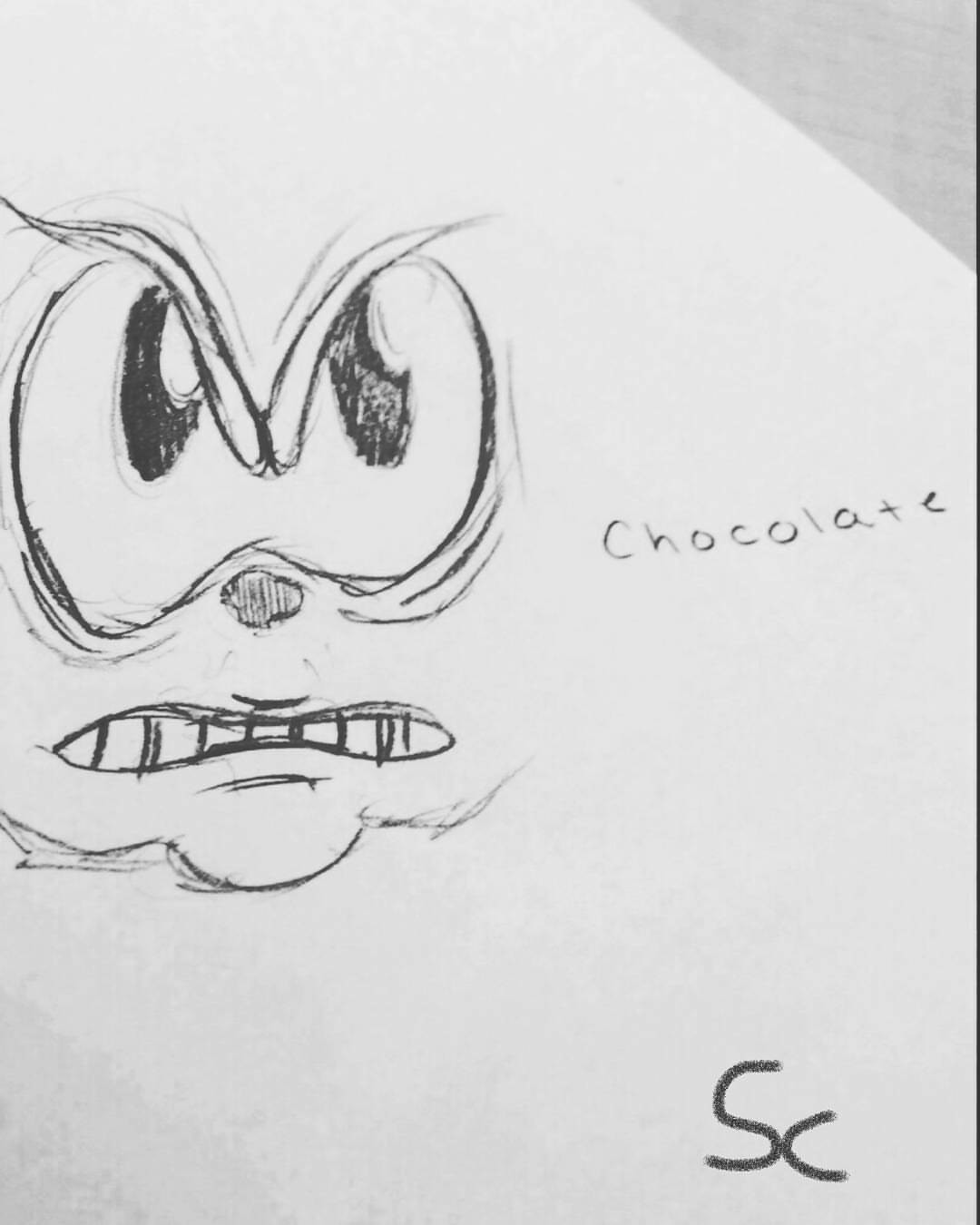A detailed sketch on a potentially white sheet of paper or an indistinct white background dominates this image. In the top right corner, there is a faint gray shading. The central figure is a cartoon character with a menacing demeanor. This character features large, intense eyes under furrowed, sharply angled eyebrows, an expression that emphasizes its ominous intent. The nose is small, oval-shaped, and shaded, contrasting with its wide, oval grimace of a mouth that exposes a row of teeth. Just below the mouth, a cleft is subtly drawn on the chin. To the side of the character, the word "chocolate" is inscribed, though its significance is unclear. The artist has added a personal touch by signing the sketch with the initials "SC."